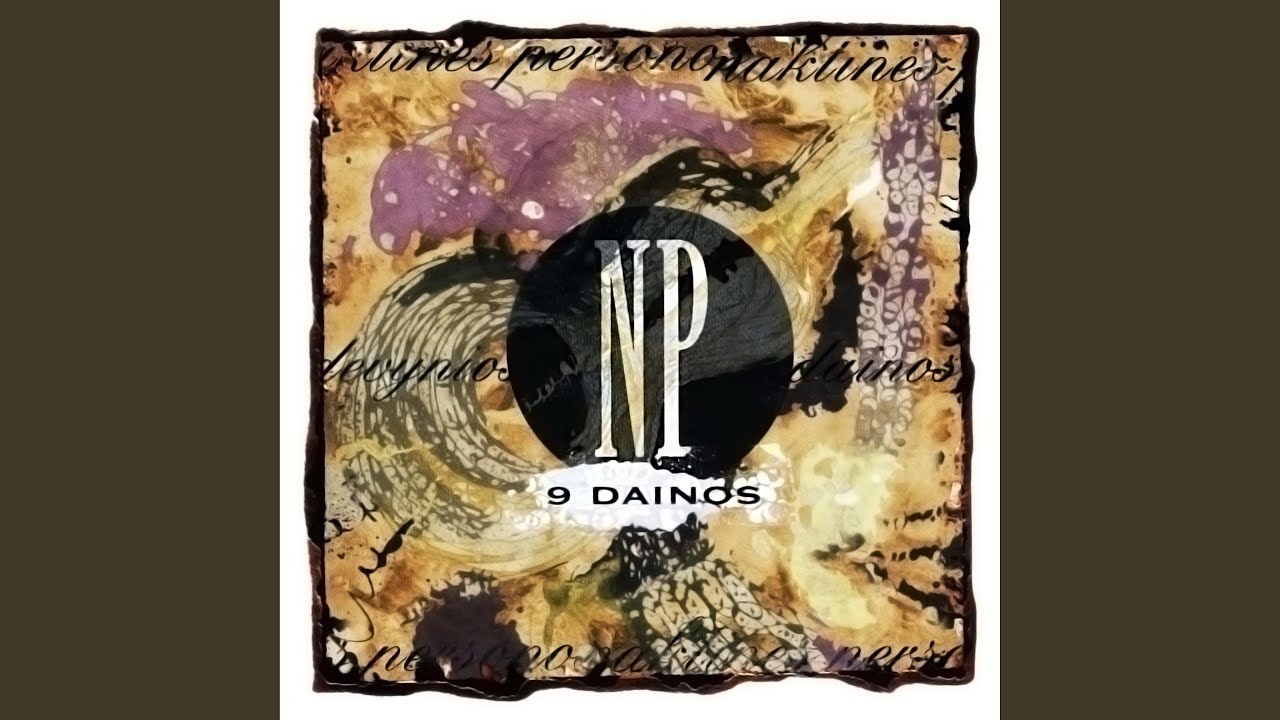The photograph appears to be a mixed-media artwork or advertisement featuring intricate details and a blend of text and imagery. The central focus is a black circle with the letters "NP" in white capitals, and below it is the phrase "9 Dainos or Danos" placed within a white cloud-like shape. This central motif is surrounded by an irregularly shaped golden and black frame, reminiscent of decal-edge paper. The artwork is bordered by two solid brown rectangles, one on each side, creating a symmetrical frame. The background features an elaborate mix of gold, black, and some purple hues, with swirling patterns and splotches that give it a batik-like appearance. The edges of the paper appear uneven, possibly shaped by heat for a unique effect. The top of the artwork includes cursive or script text that is difficult to decipher, with possible hints of words like "wines" suggesting a potential advertisement for a wine brand. Overall, the piece combines elements of text blended with the artistry, enhancing its enigmatic and abstract nature.